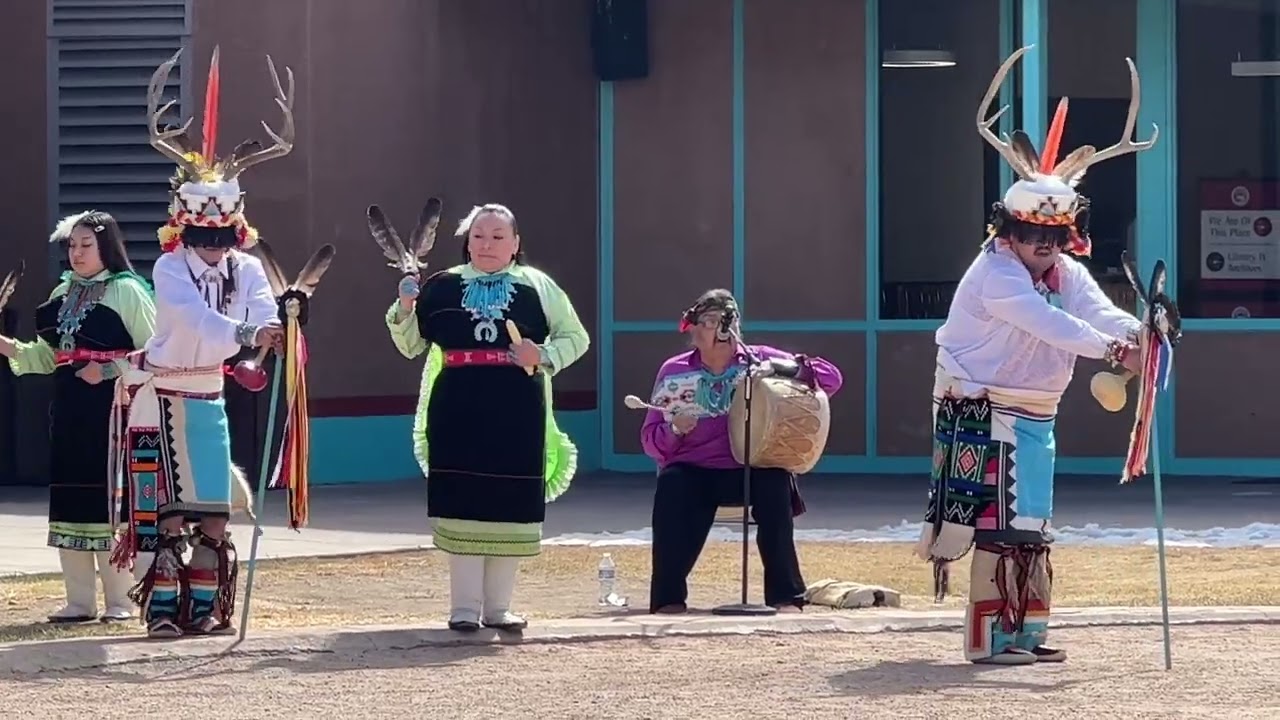This photograph captures a vibrant Native American celebration taking place outdoors in front of a tan-colored public building with turquoise trim. The scene showcases five people, all in traditional attire, engaging in a cultural performance. On the far right, a man stands out with deer antlers adorned with a prominent orange feather on his headdress. He wears a traditional outfit that includes colored skirting and ribbons. Adjacent to him, an elder gentleman in black pants and a purple shirt decorated with a design across the front is deeply involved in drumming. He holds a drum on his left knee, striking it rhythmically with a drumstick in his right hand, while singing into a microphone supported by a stand.

To the left, two women in matching black tunics with neon green long jackets and white pants stand gracefully. They both wear turquoise necklaces and white feather hair barrettes on the right side of their heads. Holding two feathers each, they emanate a sense of unity and tradition. Another man, second from the left, mirrors the attire and accessories of the man on the far right, complete with his own headdress featuring red feathers and antlers, and holding a stick decorated with long ribbons and feathers. The group is positioned on a bare ground area in front of the sidewalk, adding to the authentic and communal atmosphere of the celebration.